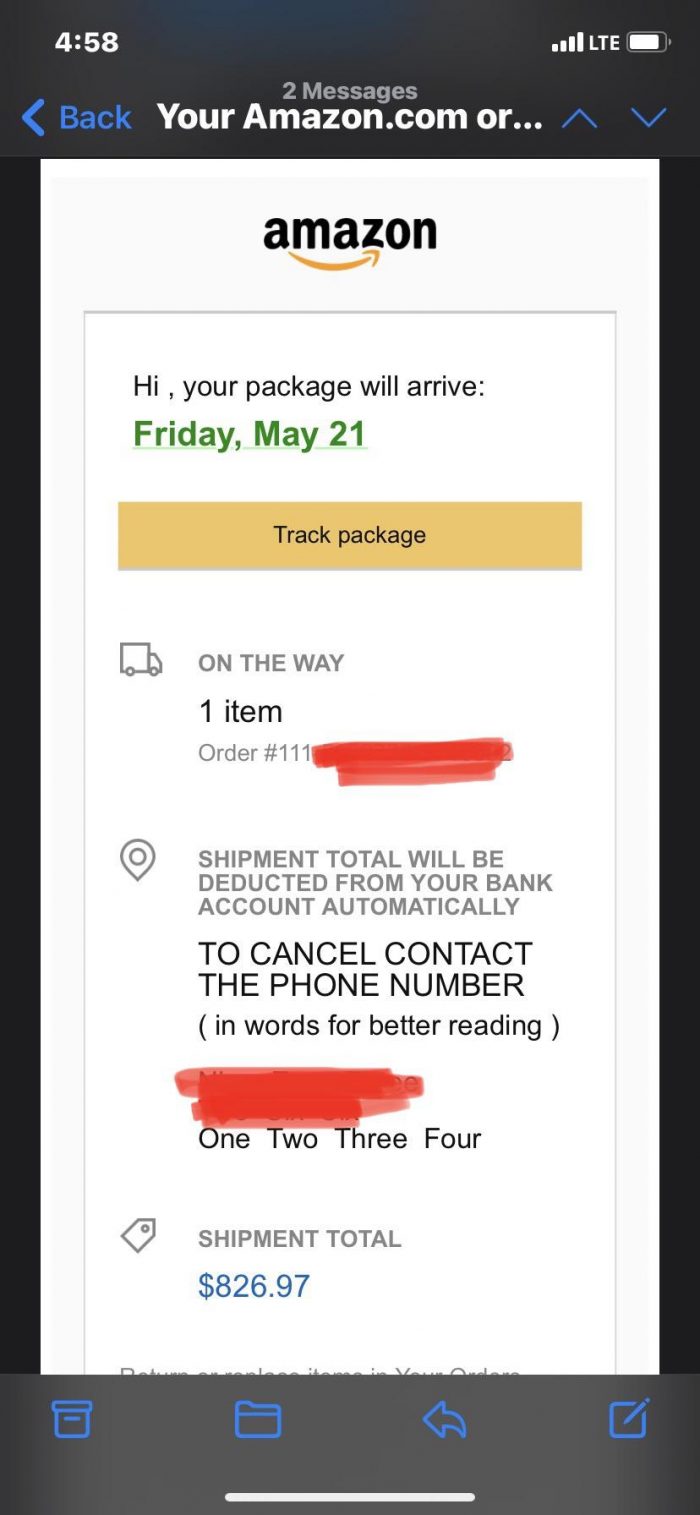This detailed screenshot from a smartphone displays various informative elements. At the top of the screen, the header bar shows the time as 4:58 (without specifying AM or PM). On the right side, it indicates full signal strength with five bars, LTE connection, and a battery level of approximately 85%, all conveyed in white icons on a black background.

At the bottom, a navigation menu with four blue icons set against a black background is visible. The icons represent: a small rectangle on top of a larger box with a line inside, a folder, a back arrow, and a classic edit icon (a square missing one corner with a pencil at a 45-degree angle).

The main content is a screenshot from Amazon.com, featuring order-tracking information. Central at the top is the Amazon logo, displayed on a gray background. Below it, a white box contains the following text: "Hi, your package will arrive" in black, and "Friday, May 21st" in green with an underline. Following this is an orange button labeled "Track Package" in black text.

Next to an icon of a delivery truck, the text states "On the way, one item, order number," with the specific order number redacted in red ink. Below this, a map location pin icon appears alongside black text that reads, "Shipment total will be deducted from your bank account automatically. To cancel, contact the phone number in words for better reading (1-2-3-4)."

Further down, a generic price tag icon is present next to the black text "Shipment total." Underneath that, the total order amount of $26.97 is shown in blue text.